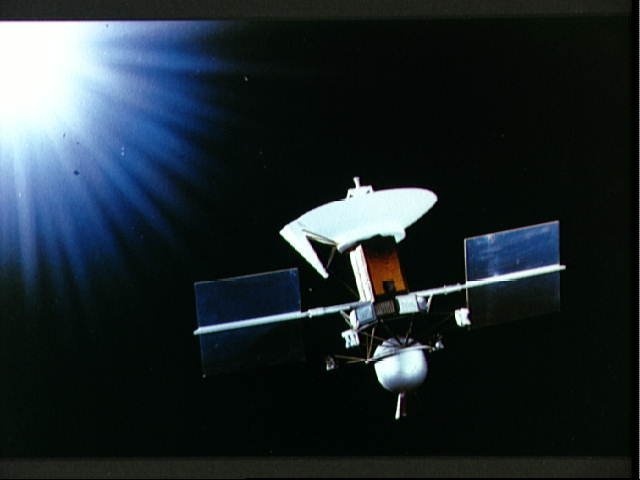The image shows a high-resolution photograph of a satellite set against the vast blackness of space, with small white dots indicating distant stars in the upper left corner. Dominating the left upper corner of the rectangular photograph, which is bordered by thin black lines at the top and bottom, is a radiant, white light, likely the Sun, emitting striking blue rays that fade from light blue to darker blue as they radiate outward. 

The satellite itself occupies the center and right portion of the image. At the top of the satellite is a white, round dish, connected to a small central box equipped with an antenna. This box is mounted on a brown rectangular body from which two metal rods extend horizontally. These rods support flat, blue rectangles on either side, which are presumably solar panels. Beneath the central box, there is a reflective silver dish.

The detailed structure of the satellite includes several distinctive elements: a conical white component near the top, a brown tubular extension, and an intricate array of shapes and connecting rods. The wingspan of the satellite features cylindrical white rods and large blue rectangular panels. Additionally, there is a gray box, a brown box, and a white box located beneath the wingspan, along with a rounded silver object that resembles the bottom of a pot. Small metal objects and a triangular-shaped horn-like structure hang from the satellite, adding to its complex design. This equipment could potentially belong to NASA or another space organization.